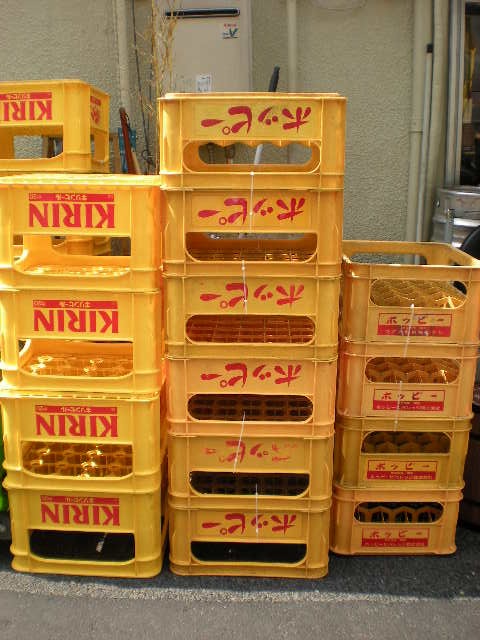This full-color outdoor photograph, taken during the daytime, showcases a series of yellow crates stacked in front of a tan-colored building with a tan door. The crates, used for carrying bottles, feature red text, including the word "Kirin" (K-I-R-I-N) prominently displayed in English alongside Asian characters, likely Japanese or Chinese. Four visible stacks of these crates are arranged in rows, with some positioned upside down. The leftmost stack consists of four crates, the central stack has six, and the rightmost stack comprises four smaller crates. The crates are set against a gray asphalt ground, with a metal keg situated in the upper right corner of the image, and the overall scene is illuminated by sunlight.